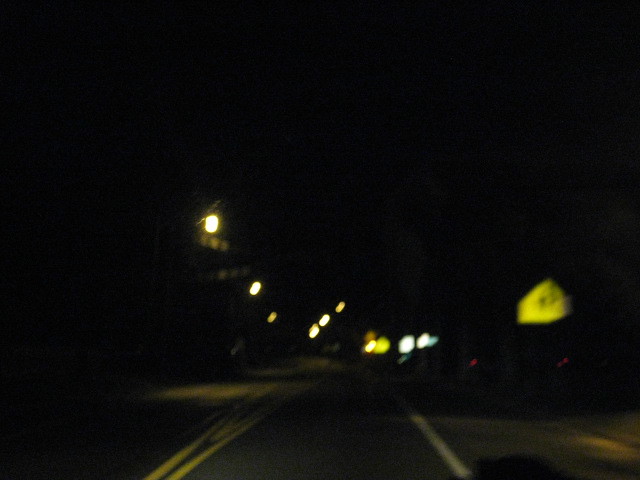Captured on a slightly blurry night, this photograph prominently features a road in the foreground. The clarity of the white line on one side and a yellow center line guide the eye down the middle of the road. On the left side of the image, a distinct yellow road sign with black figures stands out, slightly illuminated by the ambient street lights. The street lights themselves vary in color, some casting a warm amber glow, while others emit a softer, white light. In the distance, several more signs can be seen, though they appear blurry; among them are two white signs and another yellow sign, reflecting the light around. The pavement is dimly lit by the streetlights, creating a gentle glow below. In the foreground, a small black shape is visible, adding a mysterious element to the scene.